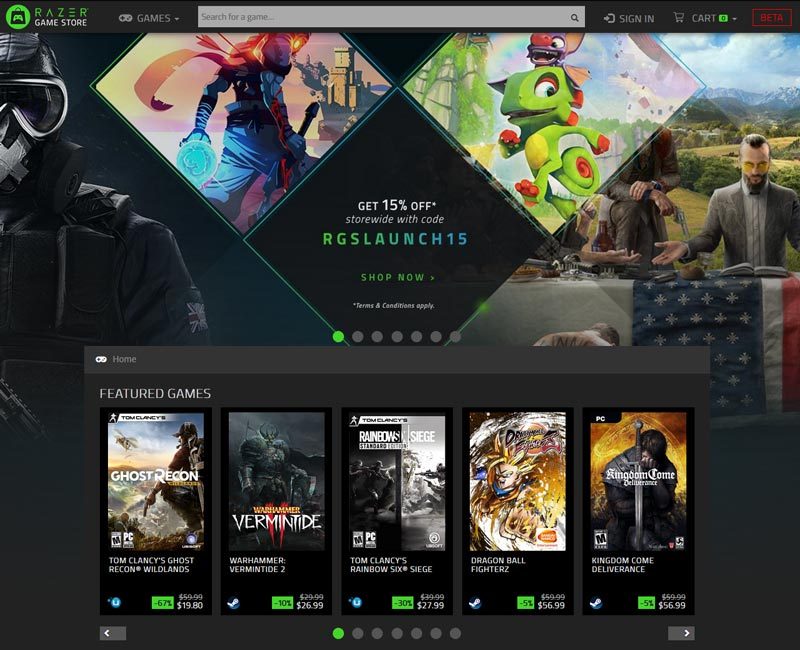The image depicts the homepage of the Razer Game Store, identifiable by the text "Razer Game Store" in the upper left-hand corner. The word "Razer" is displayed prominently in green, while "Game Store" is in all capital letters and white. Adjacent to this text is the Razer logo, which is a green emblem featuring a stylized trio of snakes, set against what appears to be a black backdrop.

To the right of the logo, there is a navigation option labeled "Games," followed by a gray search box featuring the placeholder text "Search for a game…" accompanied by an ellipsis. Across from the search box, the page displays a "Sign In" button in white text. Next to this, a cart icon is displayed with a white outline and the number "0" inside a green box, indicating an empty cart and that the user is likely not signed in.

At the very top of the page, there is a red rectangular banner marked with the word "BETA," indicating that the site may still be in a testing phase.

Towards the bottom of the page, there is a section labeled "Featured Games" in white text. This section showcases several games, each listed with their titles and prices:
- "Ghost Recon" at $19.80 (on sale)
- "Warhammer: Vermintide 2" at $26.99
- "Tom Clancy's Rainbow Six Siege" at $27.99
- "Dragon Ball Z" at $56.99
- "Kingdom Come: Deliverance" at $56.99

A promotional banner overlays the top background, with a black diamond shape and white text stating, "Get 15% off your next online store purchase code." Below, in varying shades of green, the code "RGSLAUNCH15" is displayed, alongside a green "Shop Now" button. Beneath this button, the text "Terms and conditions apply" is written in white.

This detailed layout gives a comprehensive overview of the Razer Game Store’s interface, the promotional offers available, and the featured games section.